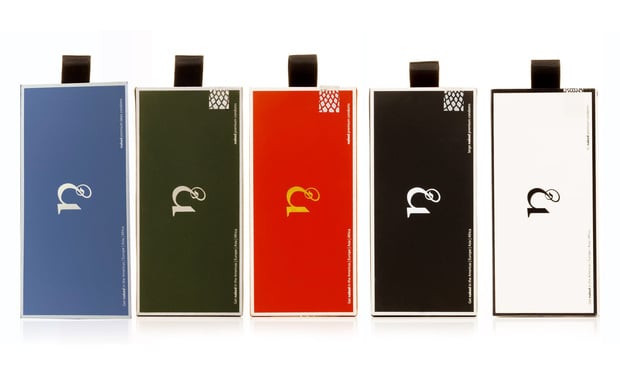The image depicts a series of five vertical rectangular bottles, likely perfume containers or flasks, each with a distinctive design and a small black cap on top. Arranged from left to right, the bottles are colored blue, green, red, black, and white. Each bottle features a central emblem resembling a sideways 'U,' with varying colors on different bottles—the blue flask has a white emblem, the green flask also features a white emblem but includes a small decorative square with black lines in the upper right corner, the red flask showcases a gold 'U' emblem and the same decorative square, the black flask has a white 'U' emblem along with the decorative square, and the white flask lacks any decorative square and displays a black 'U' emblem. The identical design of the bottles is accentuated by the color differences and the presence of the small decorative squares on the green, red, and black bottles.